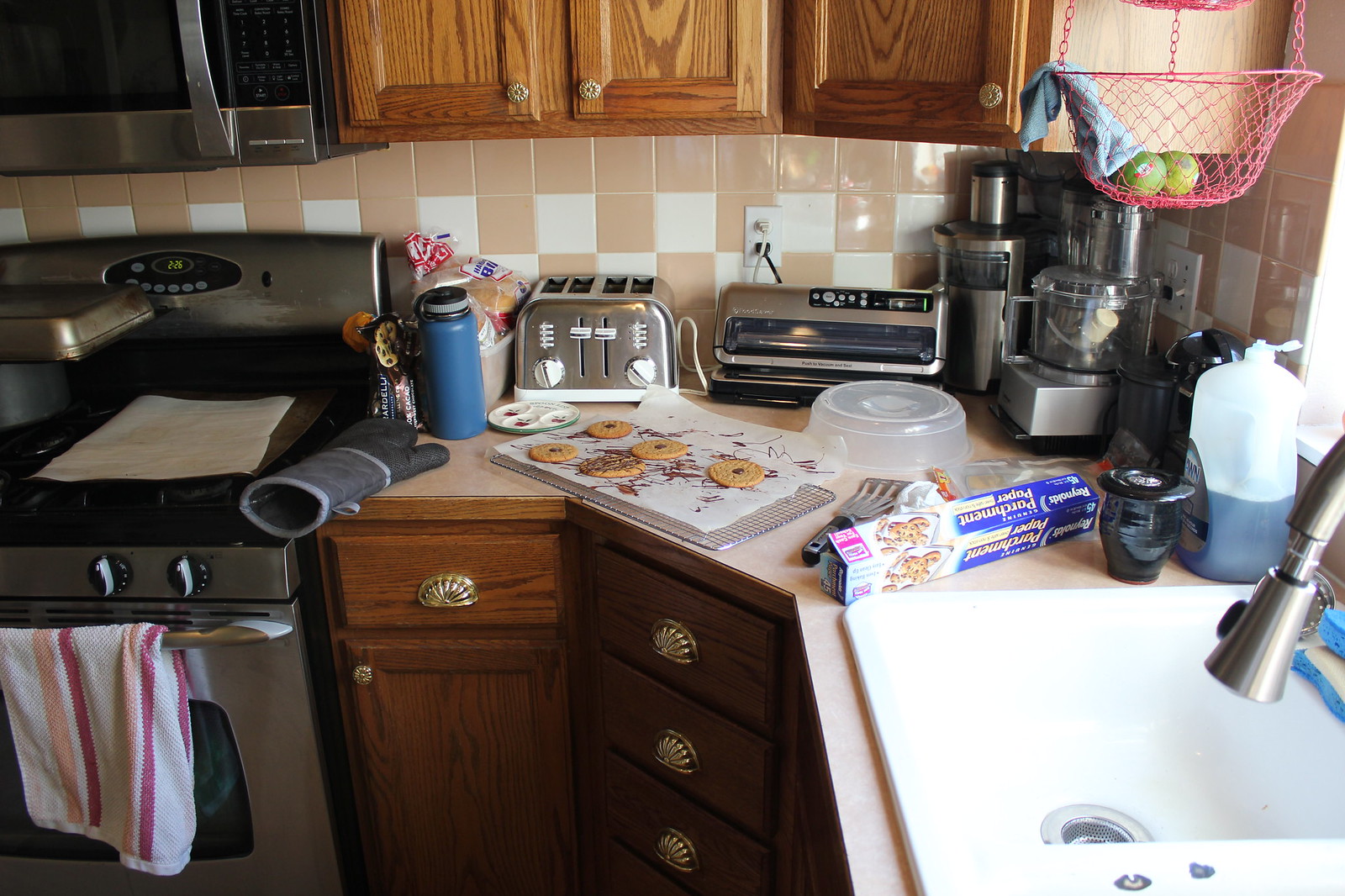The image captures a bustling kitchen corner brimming with activity as someone is in the process of baking cookies. The kitchen's backsplash features square tiles arranged in a tan and white checkerboard pattern, adding a touch of classic warmth. To the left of the frame, a sleek stove in silver and black stands out, complemented by a matching microwave mounted on the wall above it. 

Brown cabinetry, both upper and lower, frames the scene, providing a rustic contrast to the modern appliances. The right side of the image reveals a white sink equipped with a chrome or brassy telescopic arm faucet, poised for action. Next to the sink, a sandwich maker or panini press and a four-slice toaster indicate a love for varied culinary creations.

A blue cylindrical container with a black lid stands next to the stove, accompanied by a dark and light gray oven mitt, ready for handling hot trays. Nearby, a spatula, an opaque circular cover, and other shiny silver and chrome kitchen tools hint at a well-equipped cooking space. A rectangular box of Reynolds parchment paper, unmistakably blue and white, sits prominently on the counter.

Adding a splash of color, a white, orange, and red towel is draped over the stove's silver handle, its black knobs gleaming under the kitchen lights. Suspended from the ceiling in the top right corner, a pink basket overflows with bright lemons, injecting a zesty vibrance into the scene.